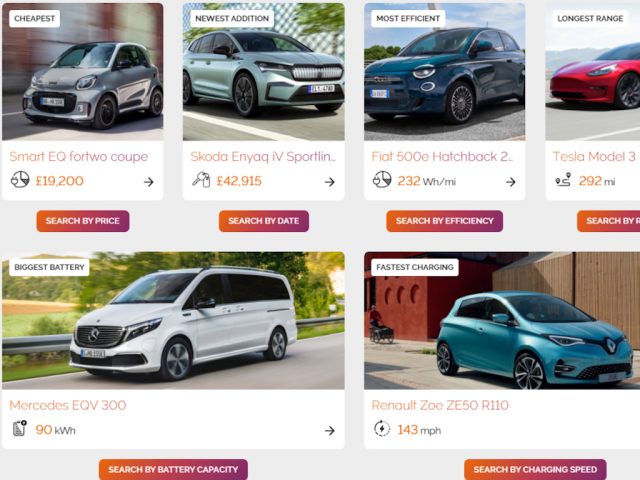The image appears to depict a car-selling website with a selection of vehicles organized in a grid layout. At the top of the page, there are four cars: 

1. **Smart EQ fortwo coupe** - Listed as the cheapest option at €19,200.
2. **Škoda Enyaq iV Sportline** - Described as the newest edition, priced at €42,915.
3. **Fiat 500e Hatchback** - Highlighted as the most efficient, offering a range of 232 miles.
4. **Tesla Model 3** - Noted for having the longest range at 292 miles.

Below these, there are two additional cars:

1. **Mercedes EQV** - Labelled as having the largest battery capacity of 99 kWh.

Between the rows of cars, there are several buttons for sorting the list, including options to "Search by Price," "Search by Date," "Search by Efficiency," and a partially cut-off button, alongside another not fully visible feature.